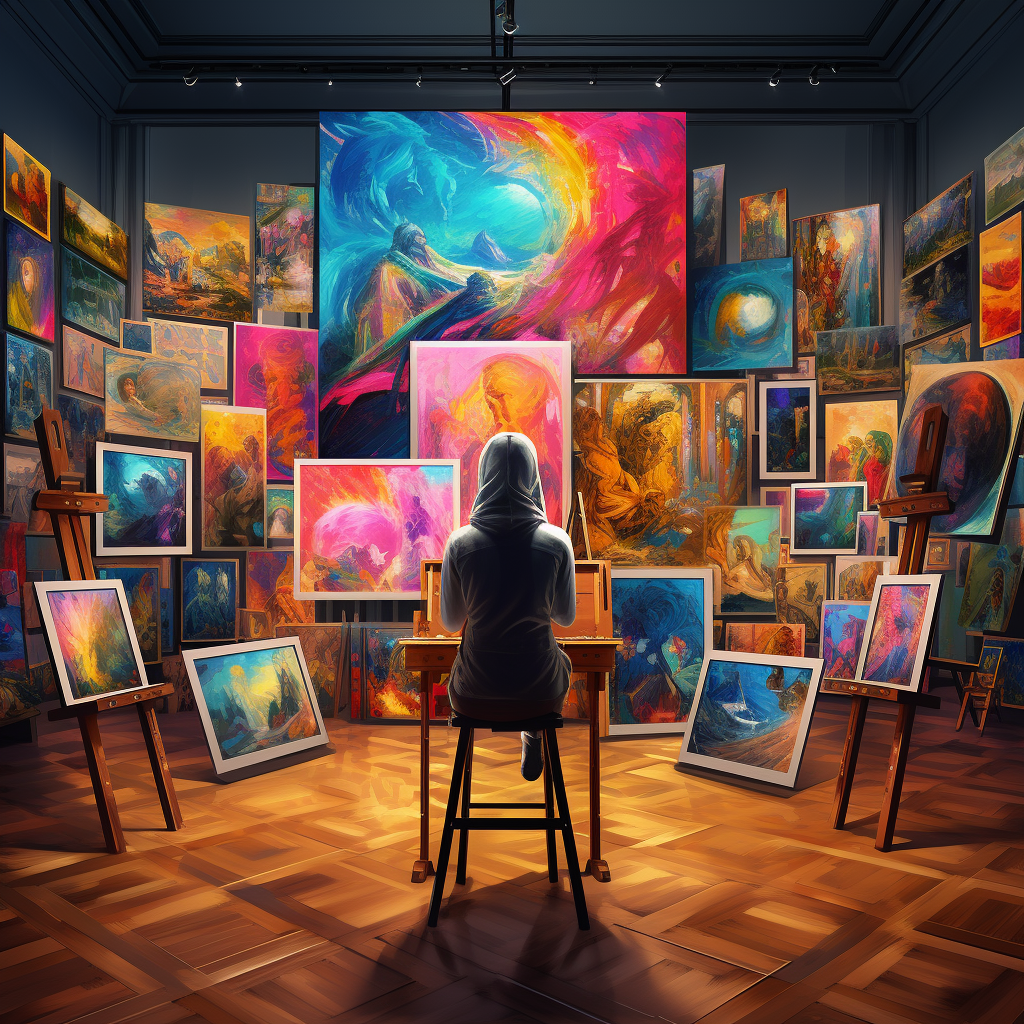The image appears to be an AI-generated or digitally animated scene depicting an artist, seated on a stool in the center of a room with a parquet wooden floor. The artist is facing away from the viewer, wearing a gray hoodie with the hood pulled up over their head, obscuring their face. They sit at a small desk or table, which is directly in front of them. The room is richly decorated with numerous vibrant paintings, covering the walls from floor to ceiling. 

To the left and right of the artist, there are easels, each holding a colorful painting. The artwork varies in size, color, and theme, with many featuring pastel colors like pink, blue, and purple. The paintings encompass a range of subjects including landscapes, oceans, skies, and abstract designs. One prominent piece directly in front of the artist depicts a dramatic scene, possibly an Indian riding a wave with fiery hues of pink and orange, while other paintings include circular patterns and underwater themes that possibly depict sea life. 

The room's dark steel gray walls provide a stark contrast to the vibrant and colorful paintings. The lighting from the front of the artist casts a shadow behind them, emphasizing their solitary figure amid the explosion of colors and artworks. This atmosphere suggests a deeply reflective and immersive artistic space.